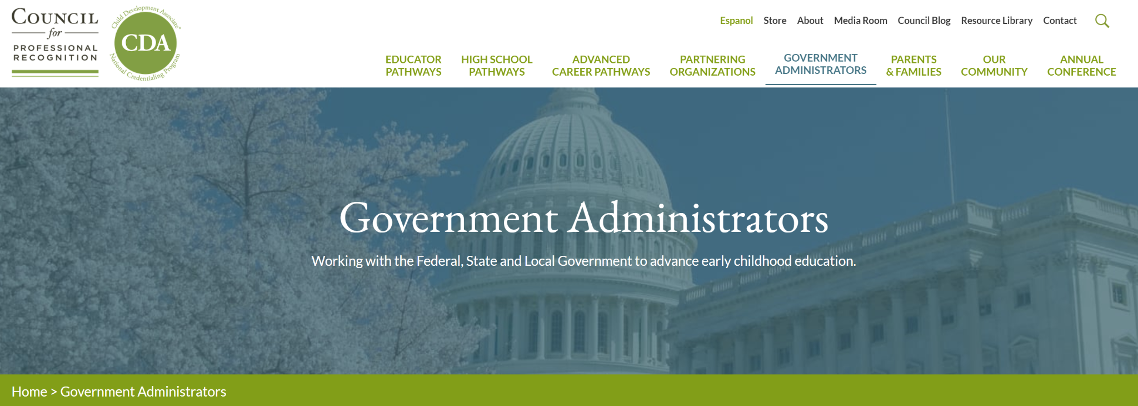This image is a detailed screenshot of an interface from the Council for Professional Recognition, prominently displaying a section dedicated to "Government Administrators." The council's logo is situated in the top left corner, presented in white text against a dark green circular background with "CDA" prominently featured next to it. The main header at the top reads "Educator Pathways," with several subpathways listed: "High School Pathways," "Advanced Career Pathways," "Partnering Organizations," "Government Administrators," "Parents and Families," "Our Community," and "Annual Conference." The "Government Administrators" section is highlighted in blue, indicating the current view.

At the very top of the page, a navigation bar provides links to "Español," "Store," "About," "Media Room," "Council Blog," "Resource Library," and "Contact." A magnifying glass icon on the top right functions as the search option.

The central section of the page prominently features the title "Government Administrators" overlaid on an image of a governmental building resembling the White House, with a subtle blue tint. On the left side of the image, there is an illustration of a white tree, adding a decorative element to the interface.